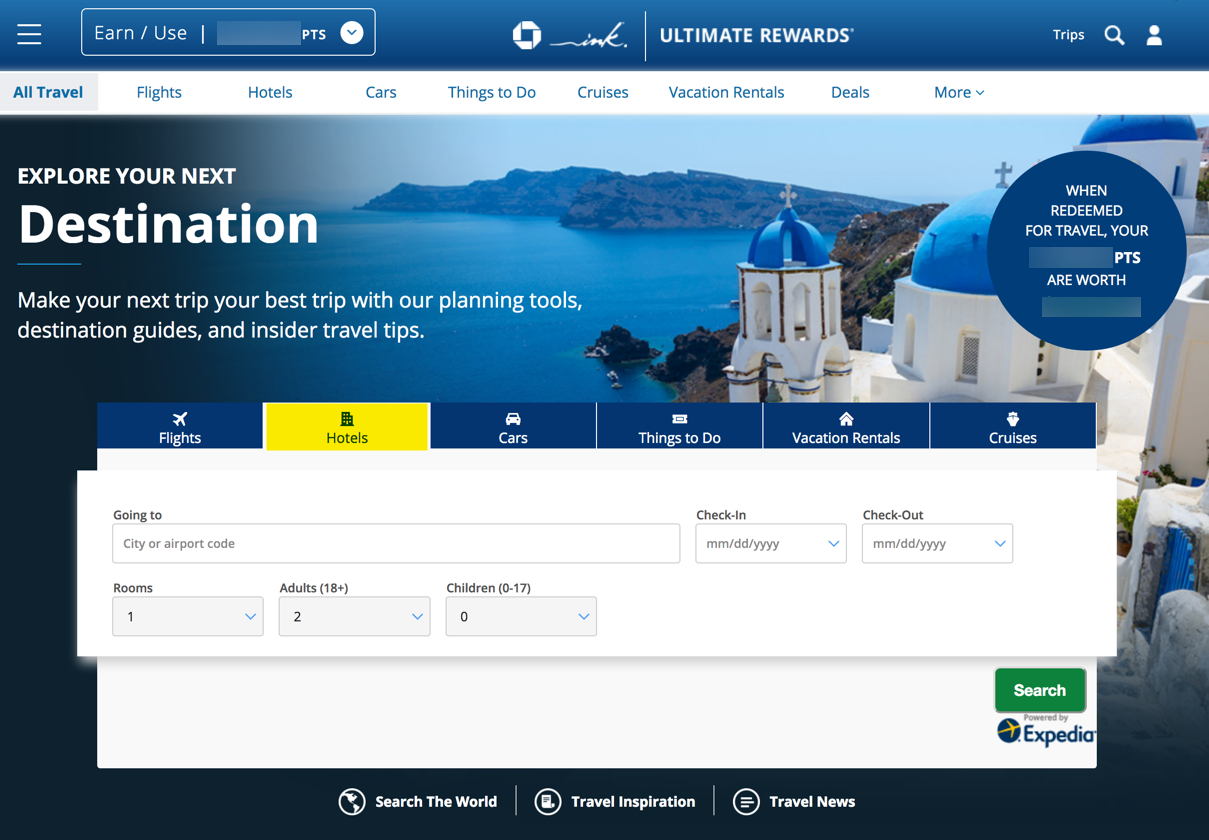A detailed caption for this image could be:

"The homepage of a comprehensive travel booking site, which allows users to book flights, hotels, cars, and other travel-related services. The interface prominently features a section where users can select hotels. You are prompted to enter details such as the city or airport, check-in and check-out dates, number of rooms, and the number of adults and children. In this instance, the form has been filled in with one room for two adults and zero children, though the dates have not been entered. 

The main background image features an ancient church, likely located in Greece, characterized by its proximity to a body of water. The church showcases traditional white-walled architecture with multiple blue domes, each topped with a crucifix. Notably, the webpage displays the Chase logo, though it is unclear if the service is directly affiliated with Chase. 

Additionally, it is mentioned that the search feature is 'powered by Expedia,' suggesting that Expedia is responsible for processing the booking details once users fill in all necessary information and click the search button."